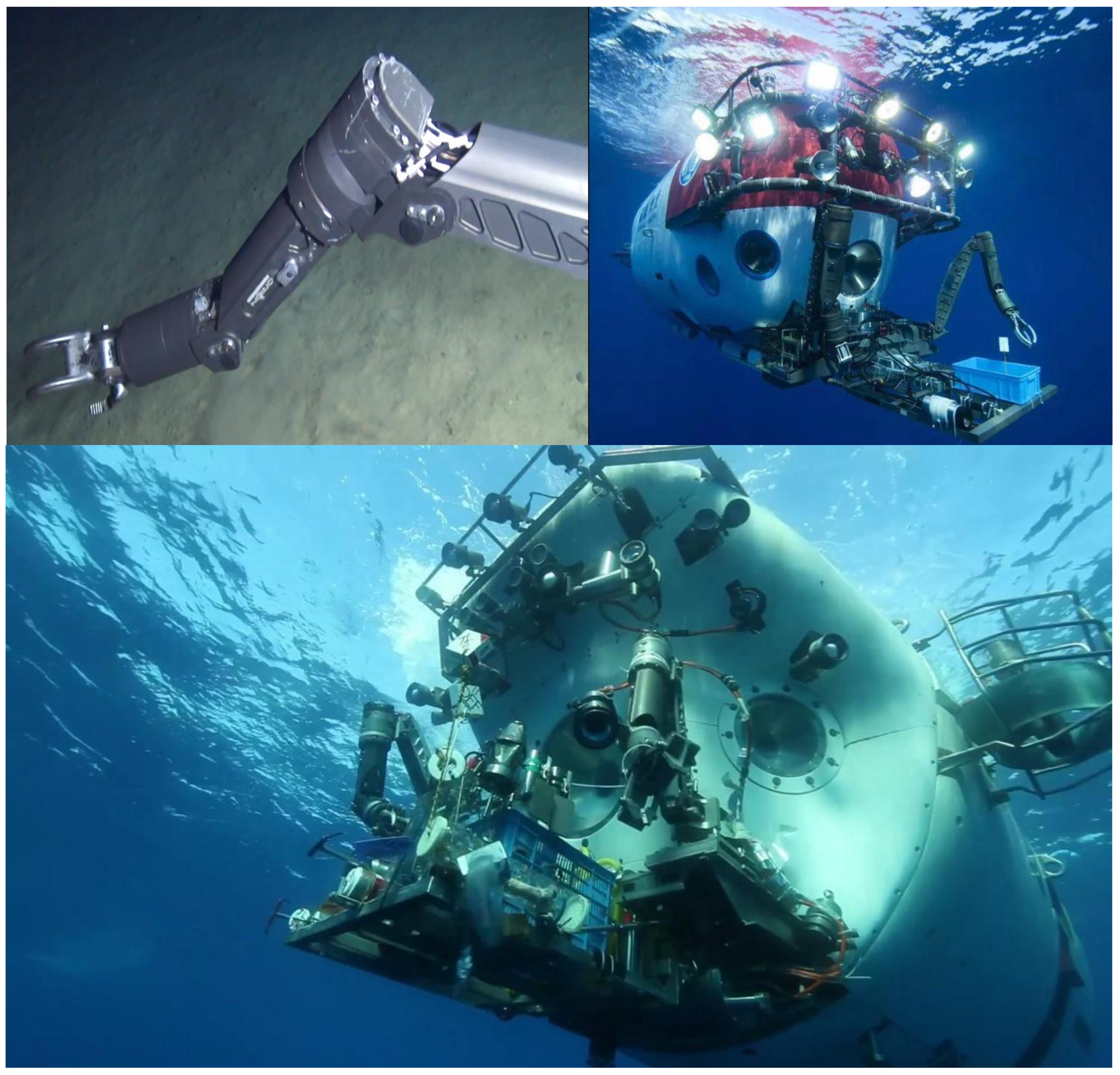This collage features three interconnected images of a sophisticated submersible vehicle. In the top-left image, we observe a black, articulated hydraulic arm equipped with clamp-like fingers, positioned near the seabed, presumably for picking up objects. The top-right image shows the rear end of the submersible partially submerged, with sunlight glistening on the water surface. This view highlights the vessel's numerous front lights and a prominent external tray likely used for storing tools. The main image on the bottom offers an undercarriage and side-angle view of the primarily white submersible, illustrating its intricate machinery and engineering. This view emphasizes three portholes – one on the front and two along the sides – as well as a large storage compartment, akin to a laundry basket, used for carrying various tools, further showcasing the vehicle's advanced design and functionality for underwater exploration and operations.